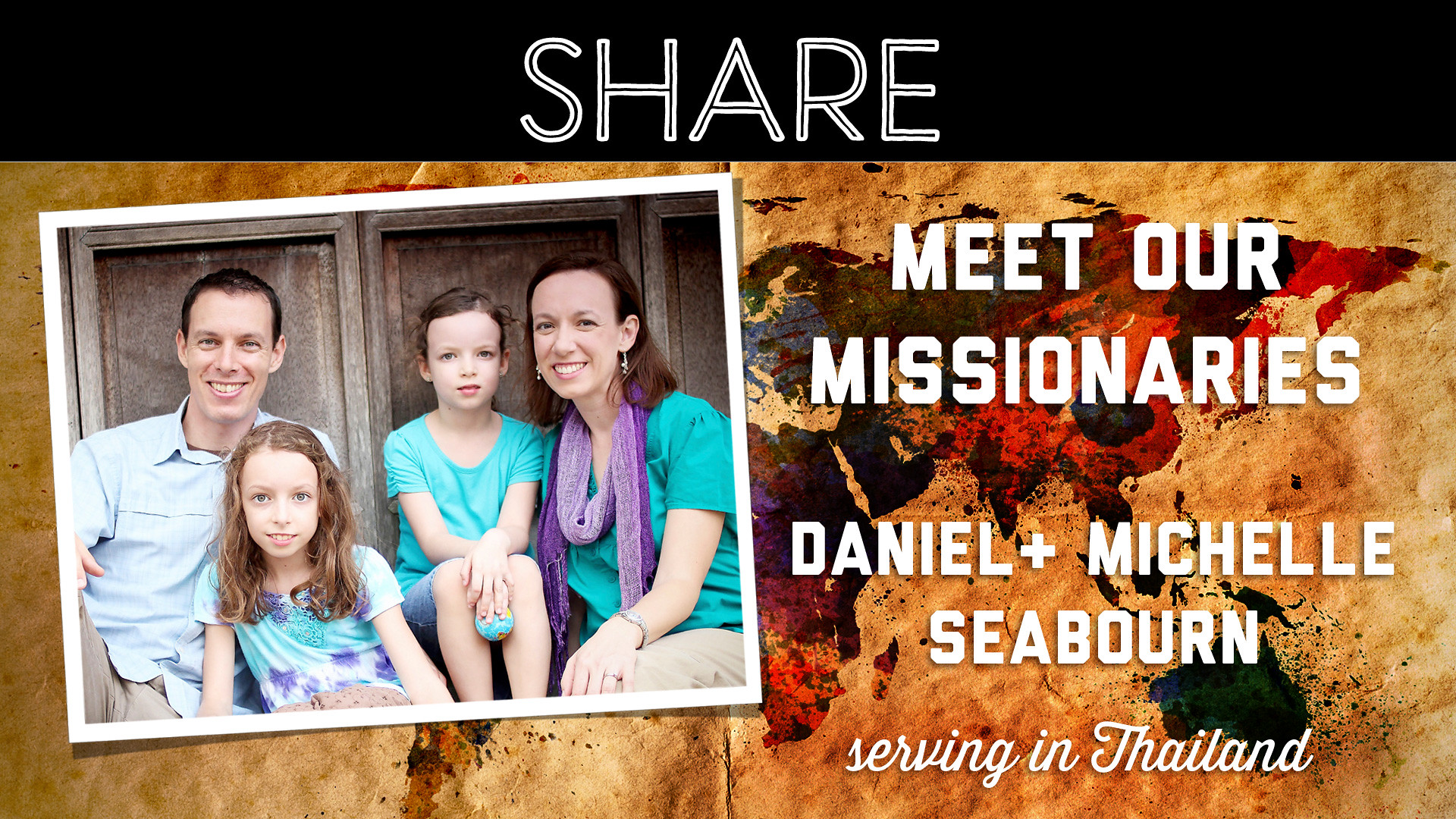The image shows a posed family portrait of four, set against a potentially ambiguous wooden backdrop, which could either be a door or a cabinet-style backdrop. The family is composed of a man with short hair, a woman with straight brown hair wearing a blue top and a purple scarf, and their two daughters, one with wavy brown hair in a blue dress and the other with her hair pulled back, also in a blue top. They are all sitting or kneeling, smiling warmly at the camera. Above the family, a black bar with white capital letters prominently says "SHARE." To the right, another section of white text reads, "MEET OUR MISSIONARIES, DANIEL AND MICHELLE SEABORNE, SERVING IN THAILAND." The background features a multi-colored map of the world, with the continents depicted in various shades resembling splashed paint, and the seas in brown and reddish-brown tones, giving it an old-paper appearance. This image seems to serve as an advertisement for the Seaborne family's missionary work in Thailand.